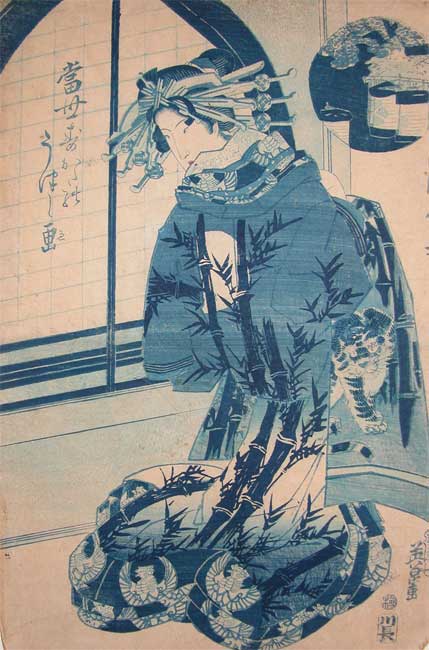The image is a detailed painting of an Asian woman, likely referencing traditional Chinese or Japanese art styles. She is kneeling on a light peach-colored surface with her knees underneath her and her arms tucked under her sleeves, pressing against her chest. Her black hair is adorned with an intricate headpiece featuring metal handles that resemble daggers. She wears a light blue dress with a decorative pattern of bamboo, leaves, and tigers. Notably, there are white circular spots on her dress near the chest and waist, resembling areas where sunlight is blocked by trees.

The setting is a traditional room indicated by the oriental details and Asian mannerisms. Behind her, to the left, stands a wall with an archway featuring a grid pattern, divided by a line down the middle. There are writings in foreign characters, possibly Chinese, on the wall. In the upper right corner of the painting, a circle contains white cups against a blue background, although the details remain indistinct. In the bottom right corner, a signature written vertically in foreign characters authenticates the artwork.